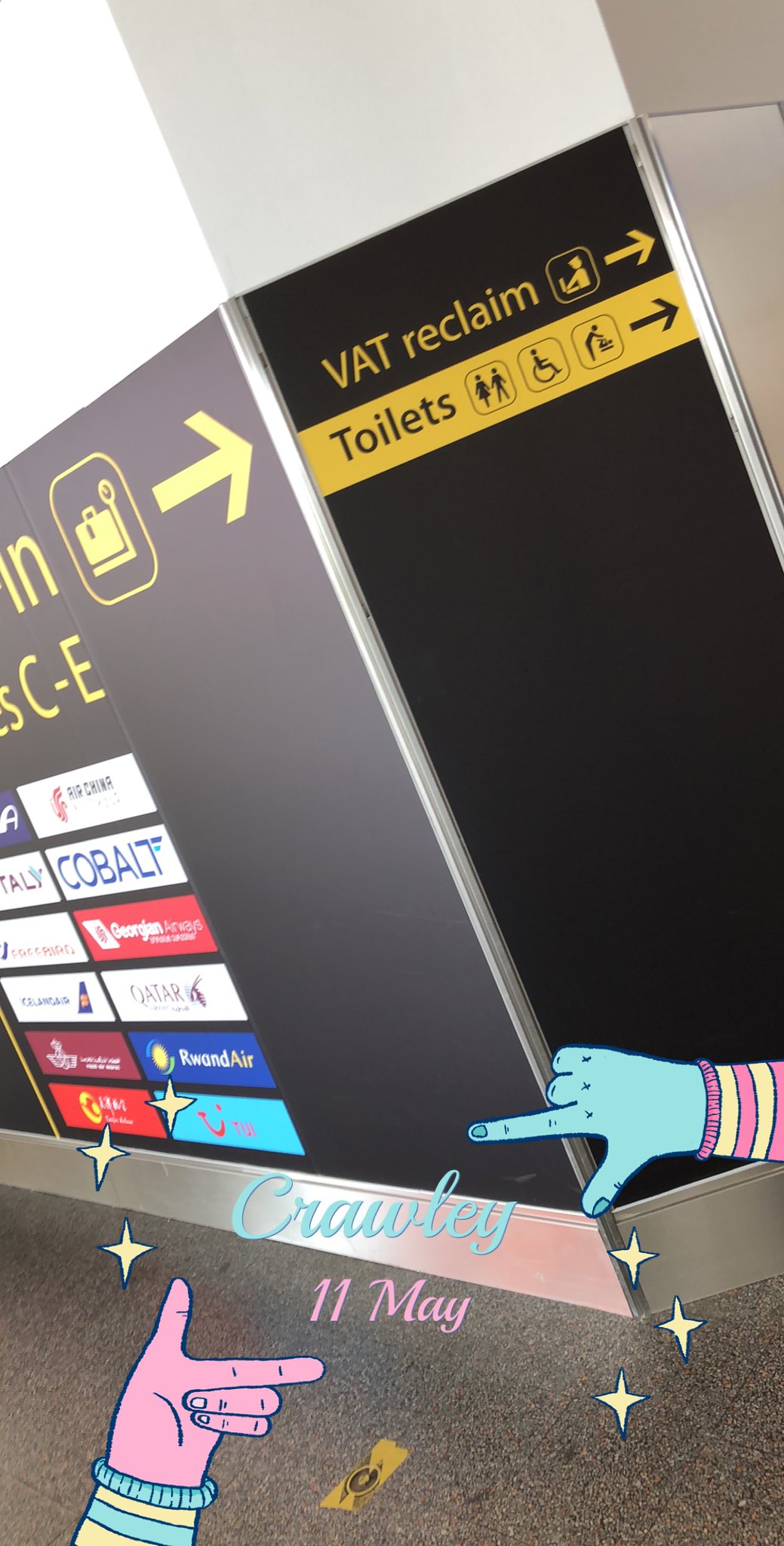The image is a screenshot of a photograph taken on a mobile phone, depicting a wall inside an airport or transportation terminal. The wall is brown and angled, adorned with various advertisements and directional signs. On the left side of the wall, an arrow in gold writing points toward the right, where the phrases "VAT Reclaim" and "Toilets" are displayed, each accompanied by arrows and icons. The advertisement for "Cobalt" is visible, although other ads are too small to discern.

In the center and bottom of the photo, a clip art overlay features two cartoonish hands making photography gestures. The left hand, positioned at the bottom left, is white with blue and white stripes on its sleeve, and has three stars ascending from it. The right hand, located toward the bottom right, is blue, wearing a pink and reddish striped sweatshirt cuff visible up to the wrist, with three stars descending from it. Between these hands, in blue font, the text "Crawley" is written, accompanied by the date "11 May" in pink font.